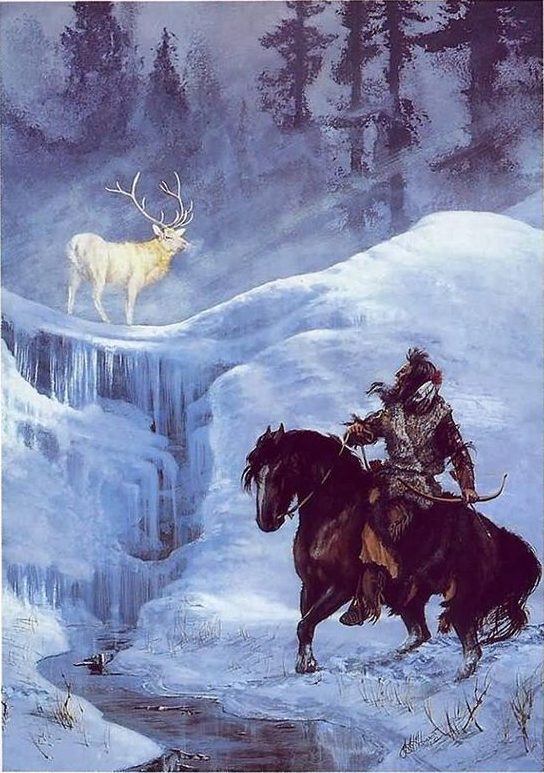In this evocative artistic illustration, we see a Native American hunter, adorned in furs with white feathers in his hair, astride a black horse on an icy hill within a snowy forest. The hunter, holding a bow and arrow in his right hand and the horse's reins in his left, gazes in awe at a majestic white elk with grand, golden antlers. The elk, bathed in a spotlight of shimmering light, stands high above on a frozen surface, looking back at the hunter. The scene captures a moment of mutual regard. The horse appears to have halted suddenly at a small, icy creek adorned with icicles, suggesting it was startled. The background features a blur of trees, further highlighting the cold and wintry atmosphere, accentuated by the flowing yet frozen creek below the elk. The entire tableau is rendered with a richness that hints at an oil painting technique.